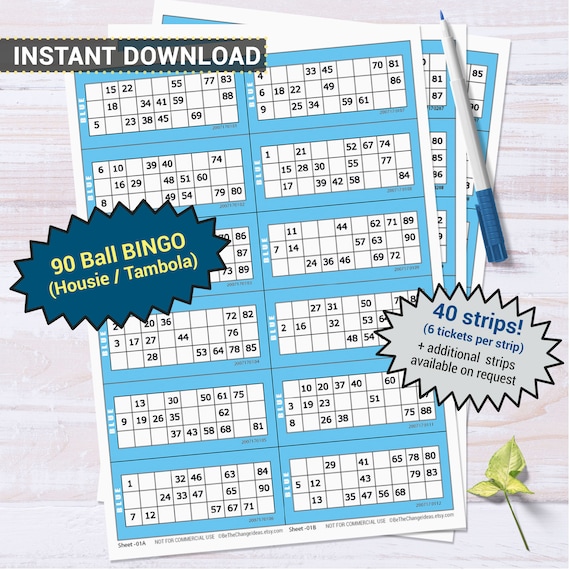This vivid advertisement features a color photograph highlighting 90-Ball Bingo Housie Tambola cards for instant download. The photo is set against a light tan wooden surface, perhaps a table. In the upper left corner, bold text announces "Instant Download," followed by a blue starburst detailing "90 ball bingo (Housie/Tambola)." Another silver starburst states, "40 strips, 6 tickets per strip, plus additional strips available on request."

The image prominently showcases the bingo cards, arranged in two attached strips, fanned out to display a total of 36 cards. Each strip holds 6 tickets, creating a visually appealing layout. The cards, light baby blue with white trims, are filled with numbers in their respective squares. A blue bingo marker pen with a gray body and blue cap rests on the second and third cards. Adding a touch of nature, a small green leaf with a stem lies in the bottom right-hand corner of the scene. This detailed presentation effectively conveys the product's features and availability in a colorful and engaging manner.